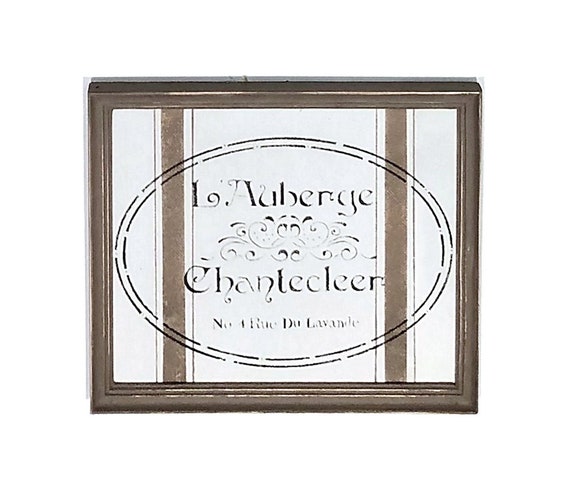The image features an aged, dark brown frame with evident wear on certain parts, suggesting its old age. This frame encloses a rectangular, shadow box-like structure, likely around one to two inches deep. The main background of the interior is white. Running vertically along either side are thick brown stripes, flanked by two thinner brown lines that add a touch of elegance. Positioned centrally is a double oval design, formed by long dashed lines that create an interrupted circle pattern. In the center of this oval design, the text "L'Auberge Chanticleer" is prominently displayed, with "L'Auberge" at the top, followed by an ornate scroll design and then "Chanticleer". Below this, in smaller and slightly harder-to-read text, is the address "Number 4, Rue du Lavande". The overall look of the sign is somewhat worn, with the broken lines of the ovals emphasizing its aged appearance.